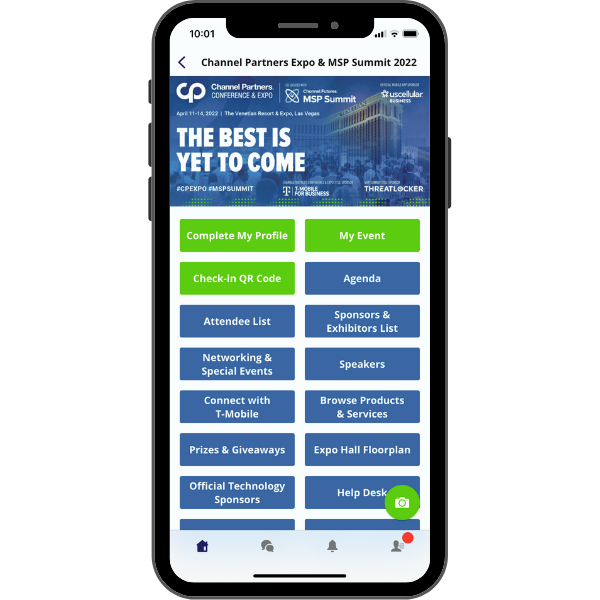This screenshot, captured on a smartphone, displays the homepage of a website. The black smartphone, outlined to emphasize the device, shows a typical interface with the top left corner indicating the time as 1:01, and the top right corner depicting a nearly full battery icon. 

At the top of the screenshot, the title "Channel Partners Expo and MSP Summit 2022" is prominently displayed in bold text. Directly below this, a blue banner stretches across the screen, featuring the text "Channel Partners Conference and Expo" on the top left, alongside a logo with interwoven letters "C" and "P," resembling an almost-infinity symbol. 

Beneath this section, the event dates "April 11th through 14th, 2022" are clearly stated, followed by the motivational tagline "The Best is Yet to Come." At the bottom of the screen, a row of buttons is visible. The first three buttons are green, labeled "Complete My Profile," "My Event," and "Check In with QR Code," contrasting with the remaining blue buttons.